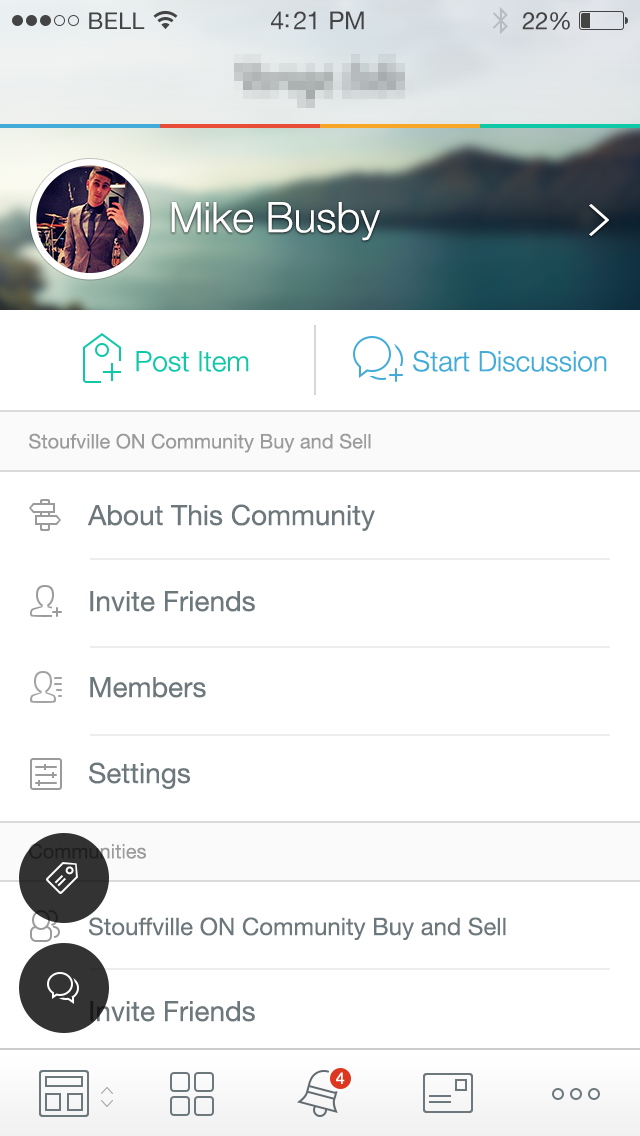Screenshot of a smartphone display showcasing a social media profile page for Mike Busby. The status bar at the top shows the network as Bell, the time as 4:21 p.m., the Bluetooth icon indicating it's off, and the battery level at 22%. Mike Busby's profile features a picture of him taking a mirror selfie, dressed in a gray suit and a black tie with short cropped hair. The page includes options for “Post Item” and “Start Discussion” specific to the "Stouffville Community Buy and Sell" group. Navigation buttons include “About this Community,” “Invite Friends,” “Members,” and “Settings.” Additionally, sections for "Stouffville Community Buy and Sell" and "Invite Friends" are present. Icons at the bottom of the screen allow for viewing in a tile layout, checking notifications (with four current notifications), accessing mail, and more settings marked by three dots. Hover icons indicating a price tag and a chat button are also visible. The website name at the top is blurred, suggesting it may be in development or testing.